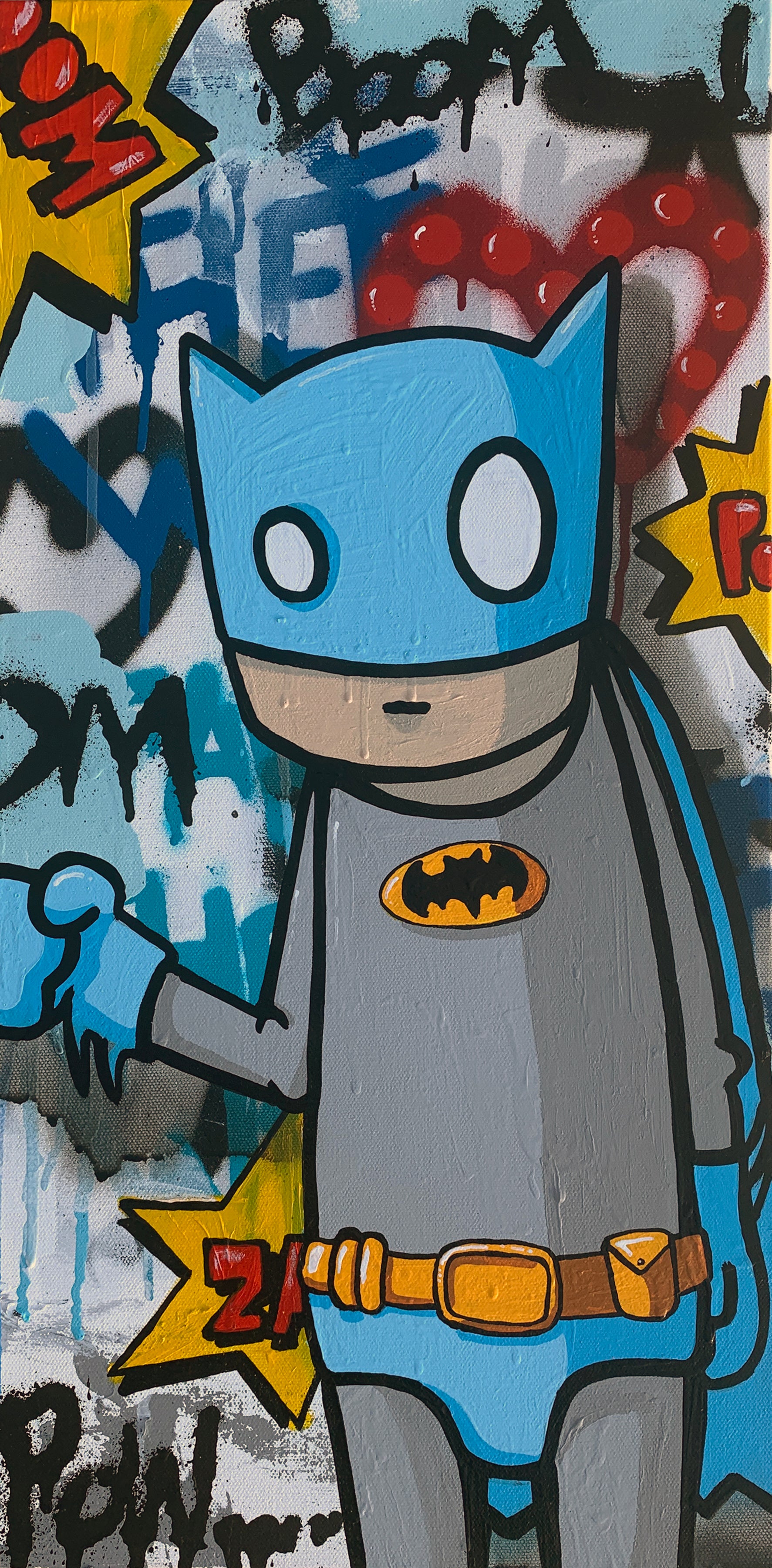This image is a color illustration of a caricatured Batman figure, executed in a graffiti-slash-cartoon style. The Batman figure stands in front of a vividly graffiti-covered wall. His attire comprises a light gray shirt and blue accessories, including a cowl, gloves, shorts, and a cape. The cowl features pointy little ears and misshapen, circular white eyes that don't align. A tiny black line serves as the mouth, and a crudely drawn bat symbol adorns the chest. A gold belt rests around his hips. The figure's blue shorts resemble a diaper due to their high-waisted fit. The background is a chaotic explosion of colorful graffiti with comic book-style action words such as "POW," "BANG," and "ZAP," rendered in bold, impactful fonts with yellow starburst effects. Additional graffiti elements include red and black hearts, and a mix of blue, gray, yellow, and red designs, completing the urban artistry.